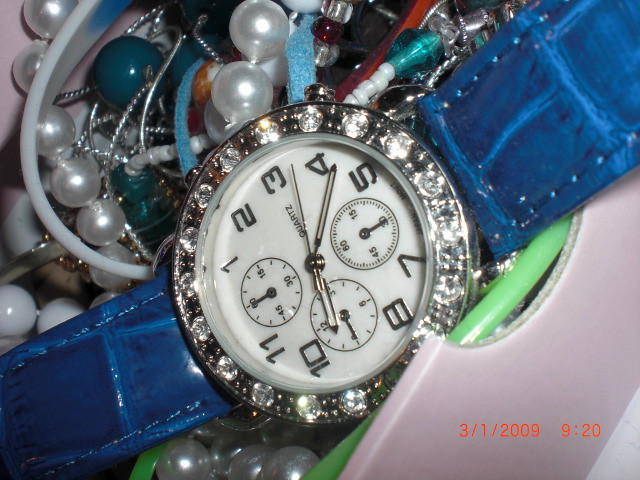This close-up color photograph, captured on March 1st, 2009 at 9:20 a.m., depicts a blue alligator skin leather strap quartz watch prominently displayed among a collection of various costume jewelry items within a container or jewelry box. The watch is positioned somewhat upside down and sideways, drawing immediate attention to its white face adorned with black numbers and three inner sub-dials indicating seconds, minutes, and hours. Surrounding the watch face are approximately 20 diamond-like embellishments set in a silver metal border. Among the scattered jewelry, notable items include white pearls and blue beads of differing sizes, along with a bracelet. A vibrant orange timestamp at the bottom right corner reads "3-1-2009-920."